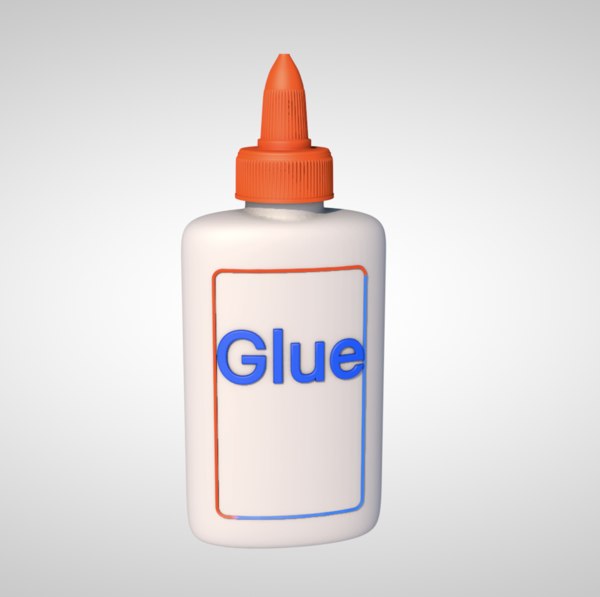The image is a computer-generated depiction of a classic, white plastic glue bottle, reminiscent of an Elmer's glue bottle commonly used by school children. The bottle stands upright and is characterized by a tall, rectangular body. The focal point is the text "GLUE," which is embossed and rendered in blue, lending a subtle 3D effect. This text is enclosed in a rectangular frame with the top halves colored in orange and the bottom half in blue, creating a distinctive border around the word. The cap of the bottle is orange, featuring vertical ridges for grip, although the very top of the cap isn’t visible as the image is slightly angled from the side. The background of the image is a gradient that transitions from a more gray hue at the top and bottom edges to a lighter gray-white in the center, providing a clean and subtle backdrop that highlights the simplicity and functionality of the glue bottle.